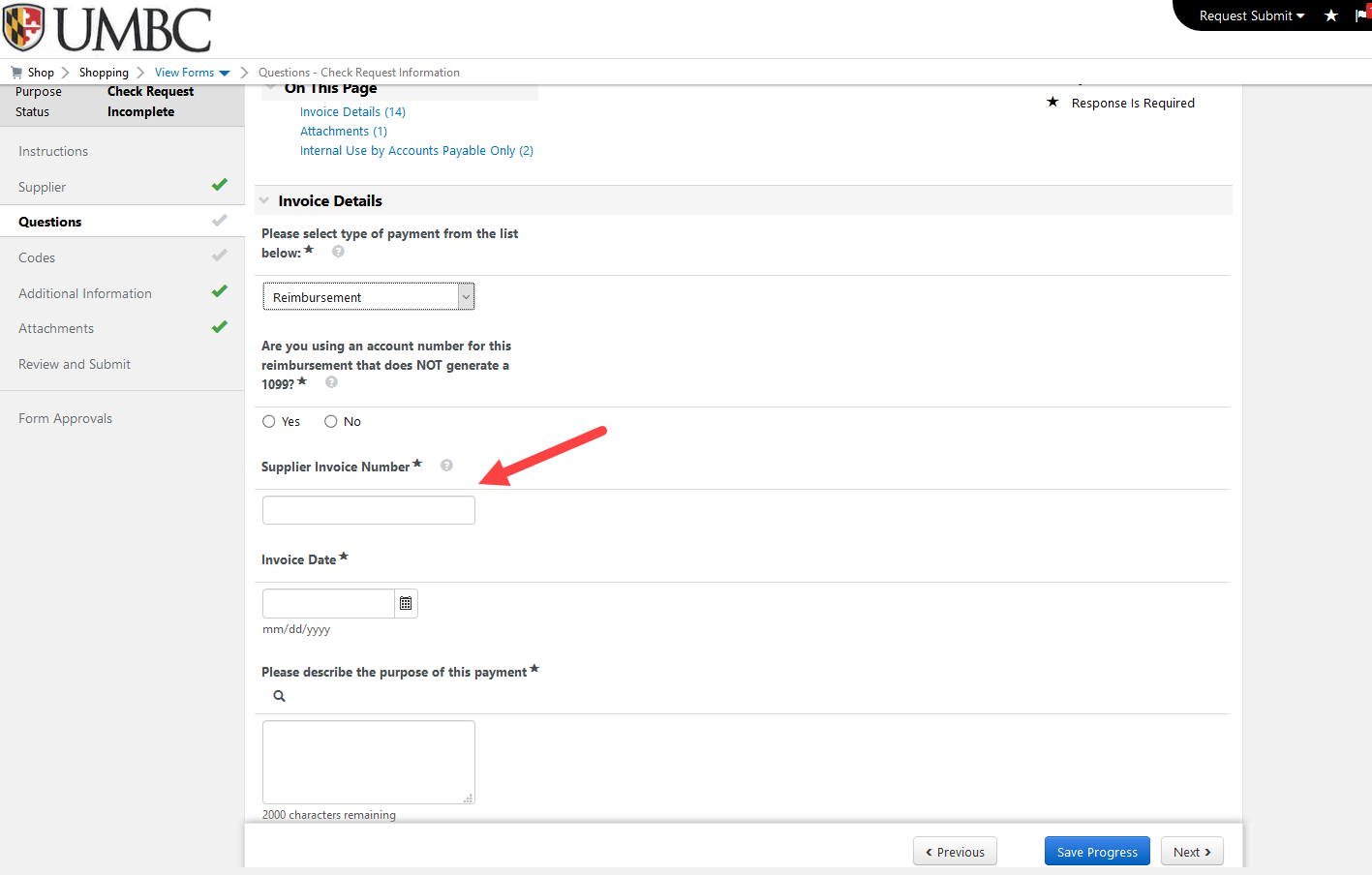**Detailed Caption for Desktop Screenshot:**

The image displays a screenshot of a desktop interface, the specifics of the browser or operating system are not apparent. At the top left, a shield emblem is visible, divided into black and yellow squares on one half, and white buildings outlined in red on the other. Adjacent to the shield, the letters "UMBC" denote the University of Maryland, Baltimore County.

To the right of the shield, the interface features a "Request Submit" button accompanied by a dropdown menu, a star icon, and a flag icon. Below this section, the options provided are "Shop," "Shopping," "View Forms," "Questions," and "Check Request Information," indicating navigational choices rather than immediate actions.

The left sidebar is aligned vertically with the headings: "Purpose," "Status," "Check Request Incomplete," "Instructions," "Supplier" (marked with a green check), "Questions" (with a grayed-out check), "Codes" (grayed-out check), "Additional Information" (green check), "Attachments" (green check), "Review and Submit" (no check), and "Form Approvals." The current active section is "Questions," highlighted for user interaction.

On the right, the primary section begins with a category labeled "On This Page" with a dropdown. The subcategories "Invoice Details (14)," "Attachments (1)," and "Internal Use by Accounts Payable Only (2)" are listed in blue text. A starred note indicates that a response is required for sections marked with an asterisk.

Within the "Invoice Details" section, users are prompted to "Please select the type of payment from the list below," where currently "Reimbursement" is selected. The form further inquires, "Are you using an account number for this reimbursement that does not generate a 1099?" with options for "Yes" or "No," although no selection has been made yet.

A red arrow highlights the input field for "Supplier Invoice Number" next to a question mark icon and a text box. Users are also required to enter the "Invoice Date" in the format of month, day, and year. Another text box allows for up to 2000 characters to "Please describe the purpose of this payment."

At the bottom of the form, navigation buttons for "Previous," "Save Progress," and "Next" are provided, suggesting this interface is part of an accounting software system used by the university for financial transactions and reimbursements.